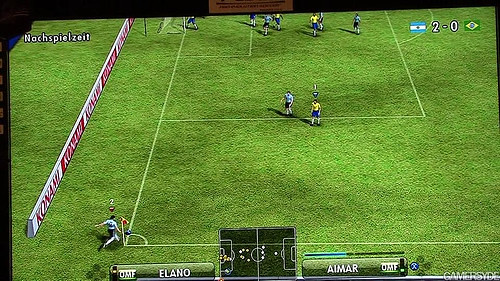The image captures an intense game of FIFA, with the lush green grass prominent at the bottom left side. In the forefront, a skilled player named Alana is actively engaged in the match. The bottom of the screen displays a field map, providing an overview of player positions. The backdrop features a wall with vibrant red and white hues, adding a sense of depth to the scene. Players in bright yellow jerseys representing Brazil and those in light blue jerseys representing Argentina are seen in mid-action. The TV screen prominently displays the score, showing Argentina leading Brazil with a score of 2-0. Additionally, the top left corner of the screen bears the match's status text, "Not Spiel," indicating that the game is in progress.